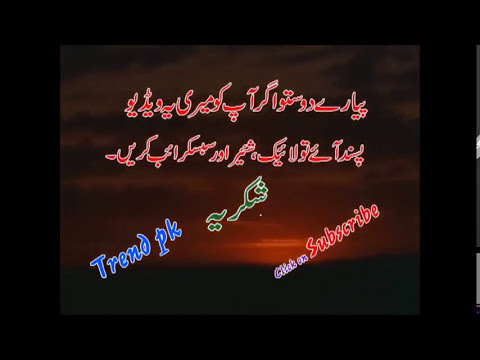The image depicts a computer or TV screen with a dark frame, capturing a hazy sky at dusk, transitioning from dark gray at the top to a warm orange near the horizon, against a thin black strip of land at the bottom. Prominent on the screen is red text in an unfamiliar language, arranged in two horizontal lines across the top half. Below this, green text in a similar script is slanted towards the upper right corner. The bottom left corner features the blue English text "Trend PK" written diagonally upward from left to right. In the bottom right corner, the command "click on subscribe" appears with "click on" in purple and "subscribe" in red, suggesting an appeal for YouTube subscriptions.